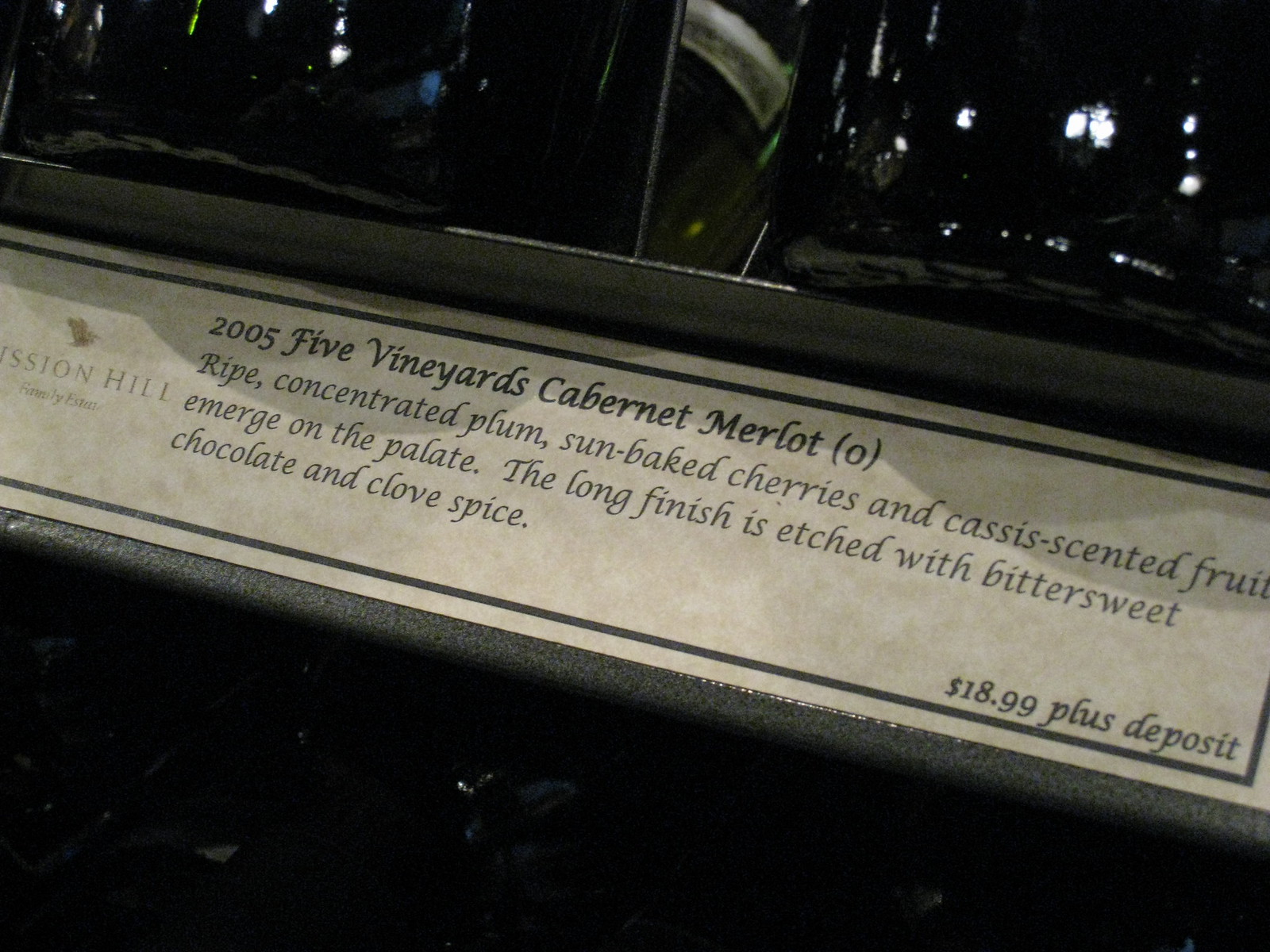This close-up image depicts a beige wine label for Mission Hill's 2005 Five Vineyards Cabernet Merlot. The label features black cursive and block lettering, elegantly bordered in black. Detailed text describes the wine’s profile, highlighting ripe, concentrated plums, sun-baked cherries, and cassis-scented fruit that emerge on the palate. It also mentions a long finish etched with bittersweet chocolate and clove spice. Positioned underneath a row of wine bottles, the label has a price tag of $18.99 plus deposit in the bottom right corner. The top line of black letters is larger than the rest, and there's a partially visible word on the left side, suggesting 'Passion Hill' with some text possibly cut off.